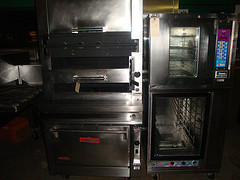This image depicts a somewhat dimly lit, indoor kitchen environment, presumably in a restaurant, showcasing various industrial-grade cooking appliances predominantly of stainless steel construction. Centrally aligned are stacked ovens; the lower one, a large unit with a prominent silver handle and a red name tag across the top. Above it is an oven featuring a pull-out drawer. To the right, there are two more ovens, each fitted with glass windows and populated with wire racks designed to hold trays. The upper one presents a control panel on its right side. Throughout the image, the equipment reveals subtle highlights from a small, bright light source, likely a flash, casting reflections on their polished silver surfaces. Despite the lighting challenges and dark surrounding areas, the presence of these robust, feature-rich ovens indicates a high-capacity, professional kitchen setting.